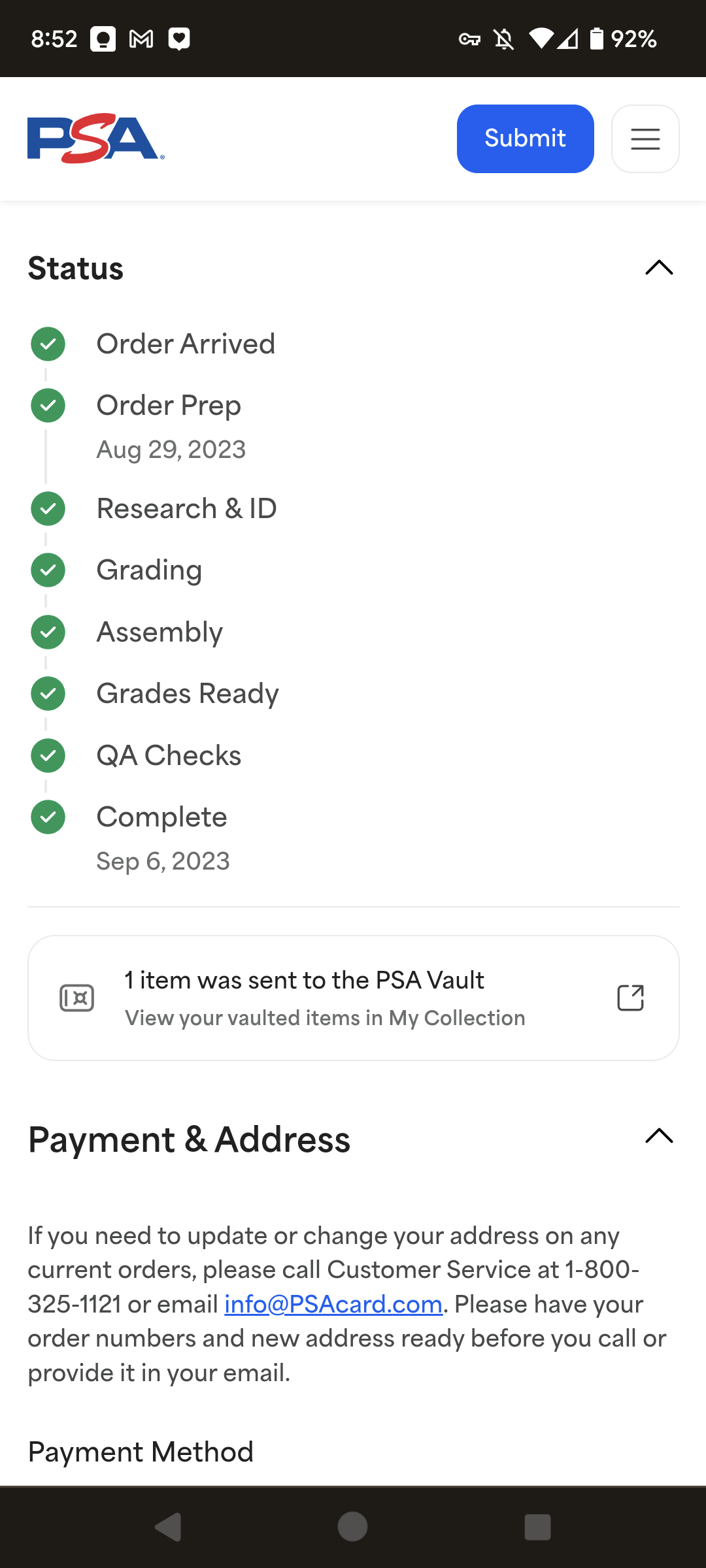A detailed smartphone screenshot displays various icons and information. The bottom black border contains a timestamp reading "8:52". From left to right, there's a light bulb icon, an email icon, a "like" icon, a skeleton key icon, a crossed-out sound icon, a strong Wi-Fi signal icon, and a battery icon showing 92% charge. Below this row, a light gray section reads "PSA" followed by a blue "Submit" button and a hamburger menu icon.

In the middle section, "Status" is displayed with an opened drop-down arrow next to it. A vertical list in green circles with white check marks includes statuses in descending order: "Order arrived," "Order prep - August 29, 2023," "Research and ID," "Grading," "Assembly," "Grades ready," "QA checks complete - September 6, 2023." 

A thin gray line separates this from a boxed section containing various square icons and the message, "One item was sent to the PSA vault. View your vaulted items in My Collection."

Below this, there's another drop-down section for "Payment and Address Details." It instructs users needing to update their address on current orders to call customer service at 1-800-325-1121 or email info@PSACard.com, providing their order numbers and new address.

Finally, the bottom border includes a left-facing arrow, a home button, and a stop button.